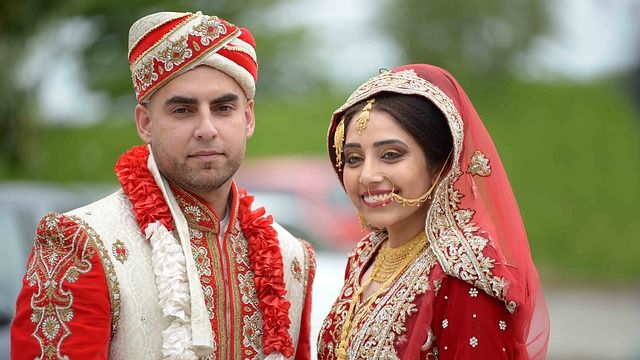A photograph taken outdoors during the daytime captures a young, ethnically Indian couple, possibly bride and groom, dressed in traditional clothing amidst a backdrop of vibrant green leaves. The woman's face radiates joy, marked by a broad, genuine smile. She is adorned in a red dress embroidered lavishly with gold designs and a transparent red scarf edged with gold applique. She accessorizes with a red and gold headband or shroud that covers her black hair, gold jewelry including necklaces, a medallion hanging down her forehead, and a gold chain that connects a nose piercing to her ear. Her intricate attire is complemented by a gold chain running from her nostril to her ear and an abundance of gold detailing.

In contrast, the man stands to her left with a noticeably stern expression, his mouth set in a thin line, suggesting that he is either upset or deep in thought. He wears a traditional red and white tunic with a red collar and gold applique on the sleeves. His head is adorned with a flat-topped turban with horizontal red and cream stripes and a single diagonal red stripe marked by a cream-colored applique. The man's light brown skin contrasts with his neatly groomed dark black eyebrows and a five o'clock shadow on his chin.

Together, the couple's elegant and elaborate attire suggests they are attending or participating in a significant event, likely a wedding, marked by a blend of traditional cultural elements and personal emotions.